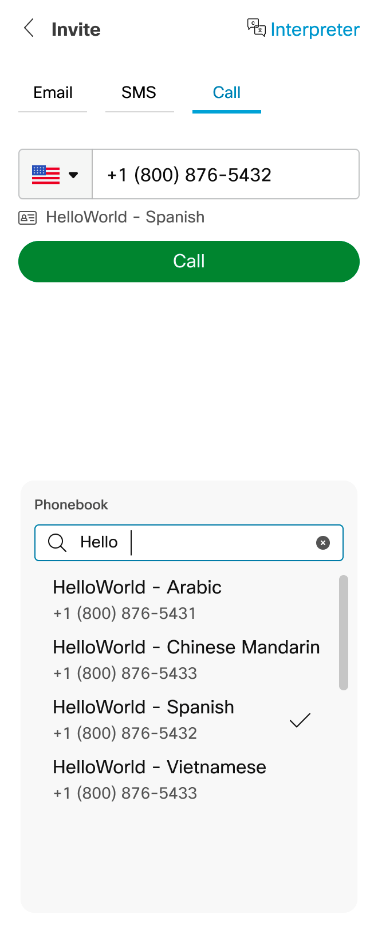This is a screenshot of an interpreter app captured from a mobile phone, evident from its portrait orientation. The background of the image is white. At the very top-left corner, there's the "Invite" text in black, accompanied by a backwards arrow button to its left. On the right, the app's logo, featuring the word "Interpreter" in blue, is clearly visible.

Below these elements, there are three contact options: Email, SMS, and Call. The "Call" option is selected, highlighted in blue. Beneath these options is a small input box to enter a phone number, with the United States selected as the country (+1). The provided number is +1-800-876-5432.

Directly underneath, the text "Hello World Spanish" is displayed, accompanied by a call button in green. Following a brief empty space, there is a small window with a light gray background labeled "Phone Book." This section includes a search bar where the term "hello" has been entered.

The search results display:
1. "Hello World Arabic" with the number +1-800-876-5433.
2. "Hello World Chinese Mandarin" with the number +1-800-876-5433.
3. "Hello World Spanish" with the number +1-800-876-5432.
4. "Hello World Vietnamese" with the number +1-800-876-5433.